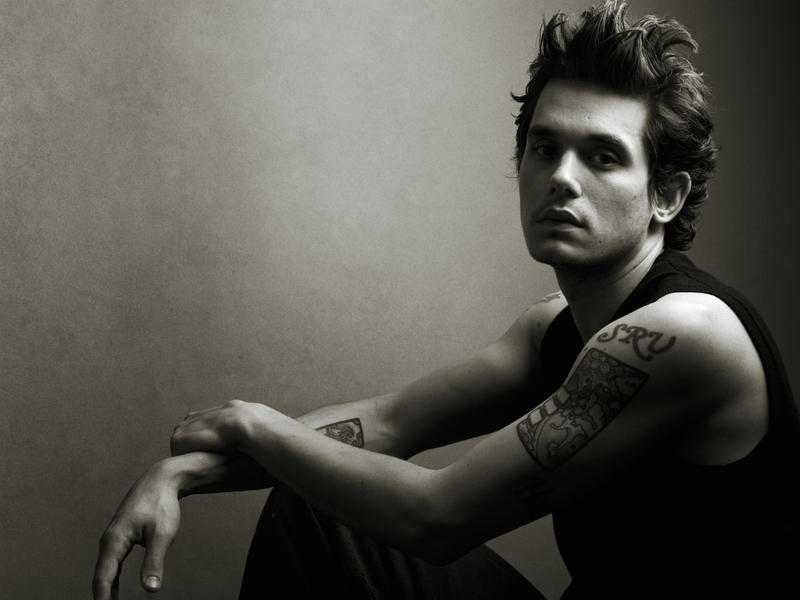In this striking black-and-white image, a man with tousled dark hair styled high on his head is captured in a contemplative, seated pose. He is presenting as male and could be a popular musician or actor. Dressed in a sleeveless black tank top, he rests his arms on his lifted knees, showcasing two distinct tattoos. On his left arm, prominently displayed closest to the camera, is a rectangular tattoo adorned with the initials "SRV" and a pattern underneath. His right forearm features another tattoo, while there seems to be the outline of a hand tattoo on his other shoulder. The man, who is Caucasian and clean-shaven, sits against a mostly nondescript backdrop. The left side of the background is white, transitioning into darker shades of gray behind him, creating a subtle, moody atmosphere without any defining context.